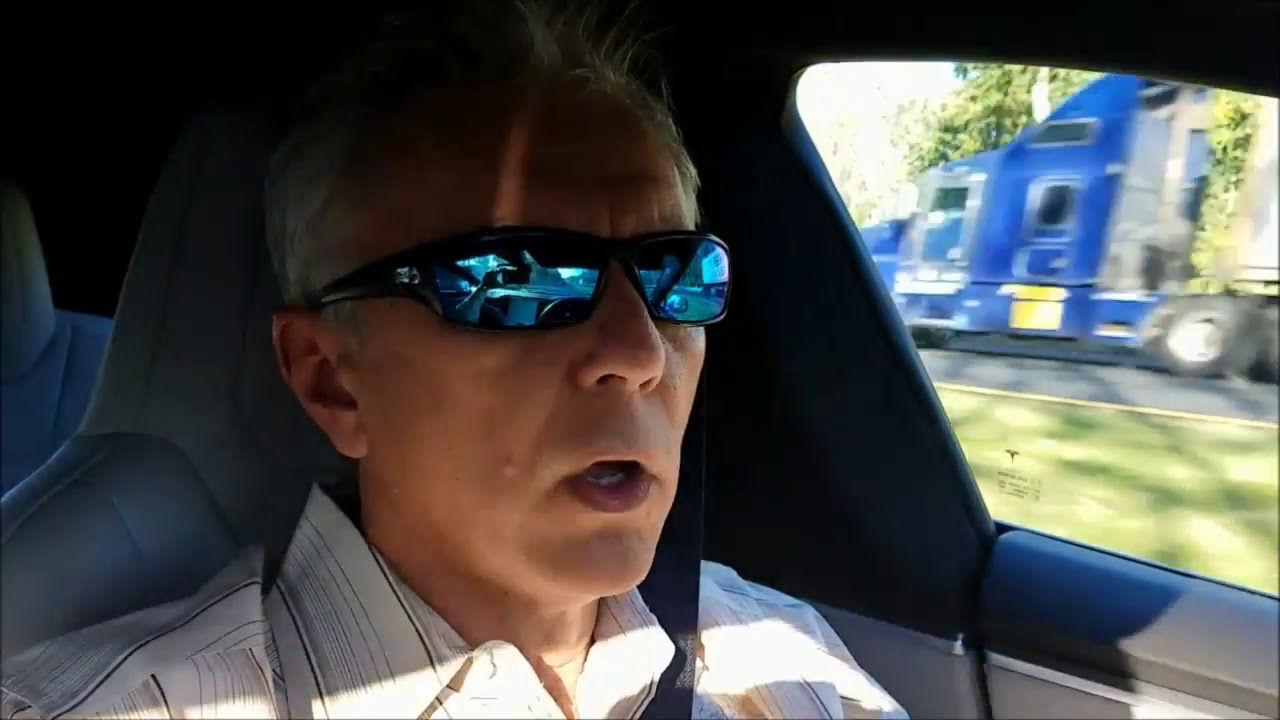The image shows an older white man with short gray hair and a partially bald head, sitting in the driver's seat of a car. He is wearing a white collared button-up shirt adorned with black and light blue stripes. His dark wraparound sunglasses, which feature shiny blue lenses, frame his face. The man's mouth is slightly open as he looks attentively at the road ahead. He is seated in a car with an interior that includes thick gray seats and a mix of dark and light gray accents. A seatbelt is securely fastened across his chest.

The setting is very bright, suggesting it is daytime. Through the driver’s side window, a blue semi-truck can be seen driving past on a road separated by a grassy median. The scene outside includes green grass and a backdrop of trees filled with lush, green leaves. The semi-truck’s deep blue cab is particularly noticeable.